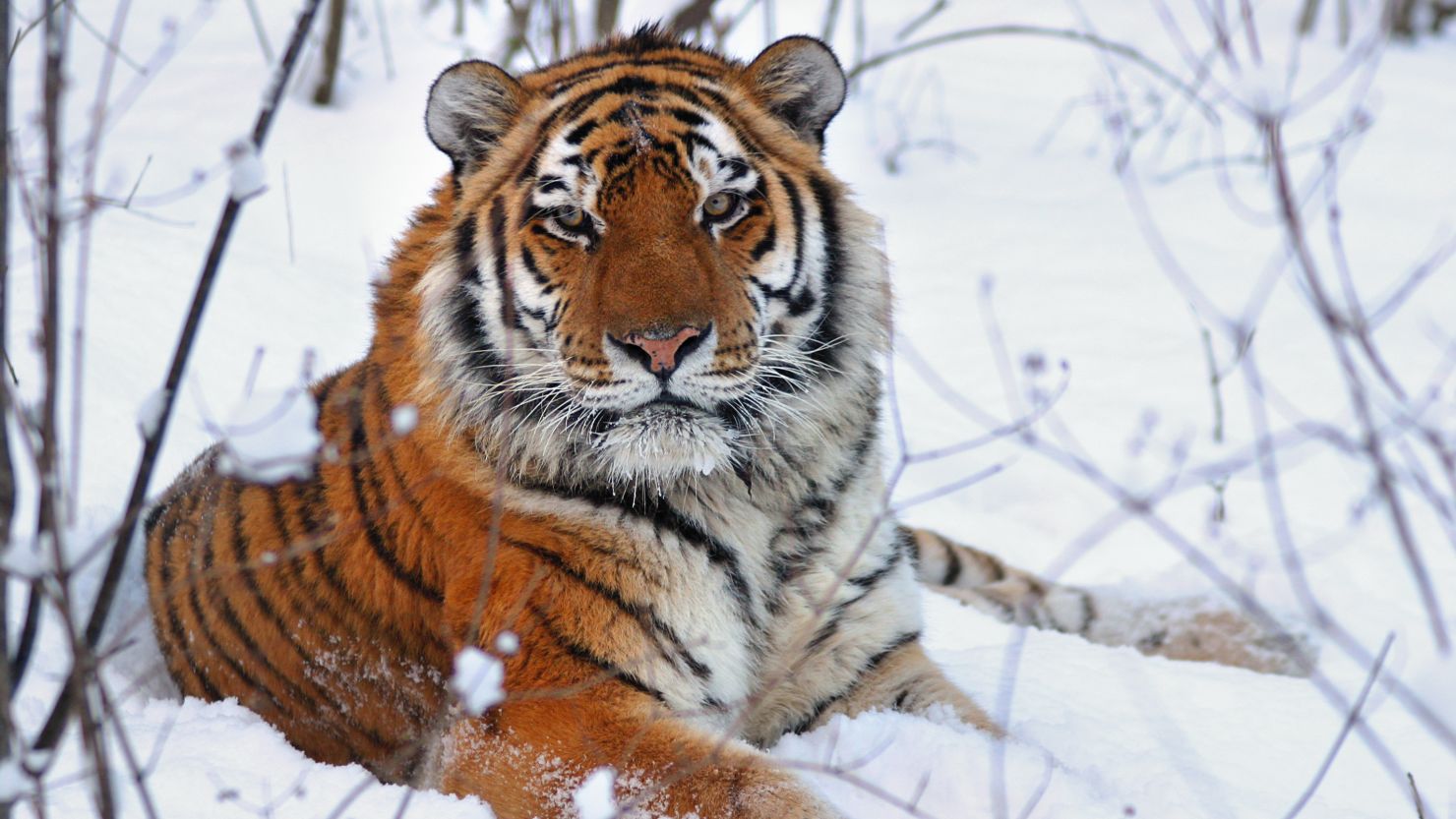In this captivating image, we see a majestic adult tiger reclining in a snowy wilderness. The tiger's robust, fluffy coat, ideal for the cold weather, boasts a striking pattern of orange and black stripes, with its white underbelly also marked by black stripes. Its face, predominantly orange, features white highlights around the eyes, mouth, and jowls, accentuating its stern expression as it gazes directly at the viewer. The tiger's yellowish-hazel eyes, with pinpoint pupils, add to its intense stare. The scene is dotted with branches and bushes, hinting at the tiger’s natural habitat. The snow-covered ground, possibly sloping slightly, surrounds the tiger, who is partially curled with its tail visible behind. Small rounded ears stick up from its head, which also showcases a pink nose outlined in black. There is even a touch of snow clinging delicately to the fur on its chin. The overall composition captures the tiger's grace and the serene, wintry environment perfectly.